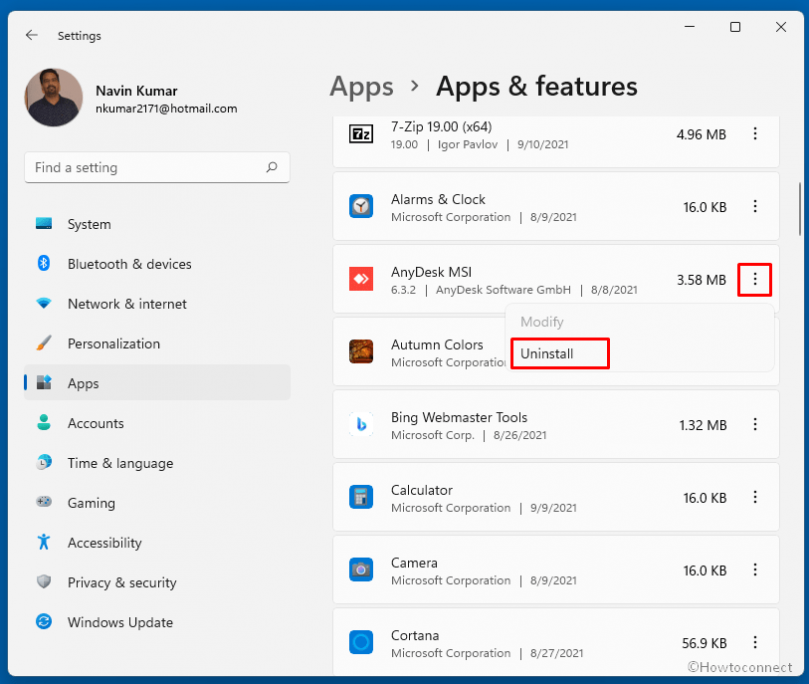An interface screenshot depicting system settings and a profile overview. On the left side, a navigation pane shows an arrow indicating a back option, followed by icons for a dash, a square, and a close (X) button. The user profile, identified as "QMAR 2171 at hotmail.com," is displayed along with various application settings.

At the top, there’s a search bar with user settings categories listed beneath it: System, Bluetooth and devices, Network and Internet, Personalization, Apps, Accounts, Time and language, Gaming, Accessibility, Privacy and security, and Windows Update. 

Highlighted software details include:
- 7-Zip 19 (64-bit) with a size of 4.96 MB.
- Alarms and Clock, sized at 16 KB.
- AnyDesk MSI, sized at 3.58 MB, which is highlighted with three vertical dots on the far right, encased in a red square.

The context menu for AnyDesk MSI shows options such as Modify or Uninstall, with the "Uninstall" option circled within a rectangle. The background showcases an "Autumn Colors" theme, providing a vibrant visual contrast to the settings text.